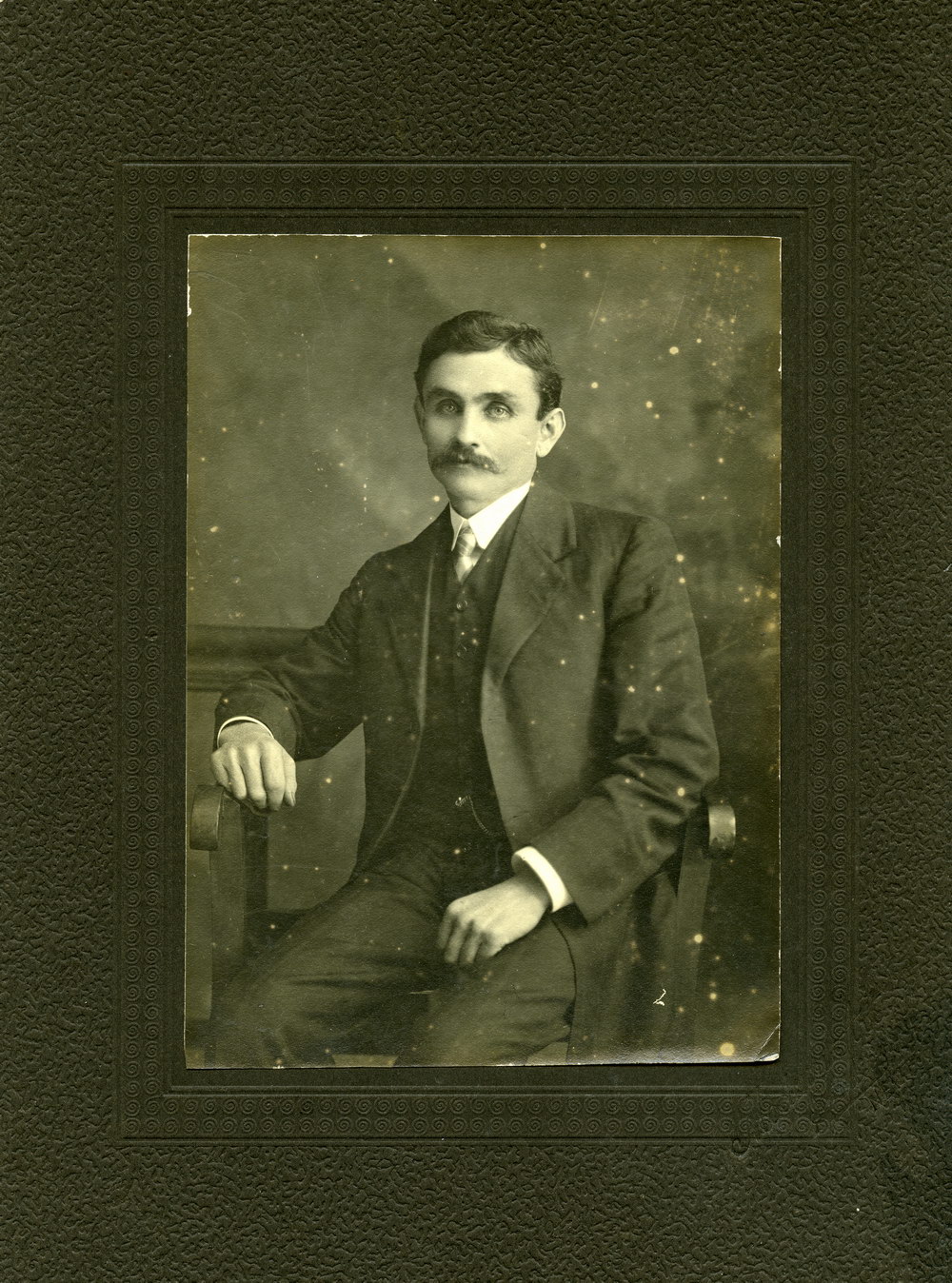A very old, vintage black-and-white photograph taken in 1911 features Michael Joseph Savage, who later became one of New Zealand's most beloved prime ministers, affectionately known as "Mickey." The slightly spotted and mildly damaged image, framed in a thick, ornate frame with swirling designs and a stippled exterior, presents Savage seated on a wooden chair. He appears to be a Caucasian male with black hair that's short and slightly wavy, and he sports a deep-set gaze with large eyes. His moustache is distinctly old-fashioned, the kind that seems almost iconic. Dressed in a suit with a long coat, vest, white shirt, tie, and suit pants, a watch fob adorns the front of his vest. Savage's right arm rests on the chair's arm while his left hand is laid on his thigh. The backdrop behind him appears to be a neutral image, perhaps mimicking clouds. The photograph, characterized by its old pose and classic attire, embodies a historical moment frozen in time.